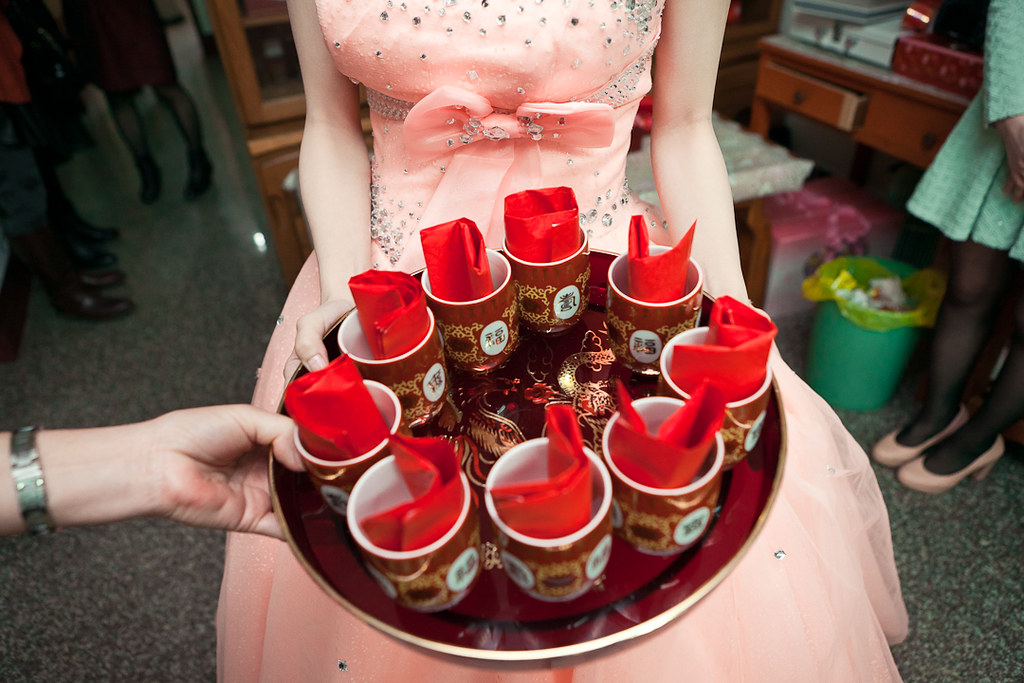In a lively party setting, a woman with very fair, almost porcelain skin, is seen holding a deep burgundy tray adorned with a gold etched dragon in the center. The tray carries nine light bronze cups, each featuring a gold design and Asian characters—possibly Mandarin or Japanese—on a white oval. Bright red napkins are neatly folded inside the cups. The woman, who appears slender, is dressed in an elegant pink ball gown with a prominent bow below the chest and extensive rhinestone embellishments on the bodice extending to the waistline. The gown is puffy at the bottom, with her bare arms bent at the elbows. Surrounding her, a woman in a green dress with black stockings and pink high-heeled shoes stands in the background, alongside other partially visible figures and a small green trash can with a yellow liner. The scene captures the essence of a vibrant celebration, rich with cultural and festive details.